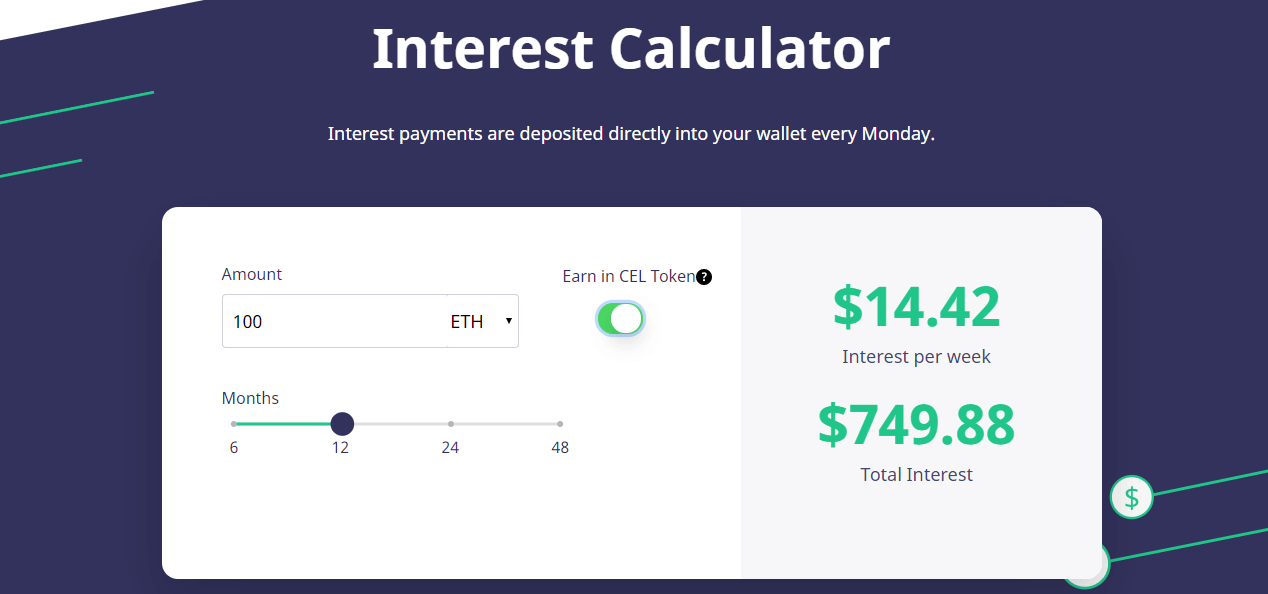The image is a detailed screenshot of an interest calculator display. At the top, the words "Interest Calculator" are prominently featured in white text. Below, a message reads "Interest payments are deposited directly into your wallet every Monday," emphasizing the regularity of the deposits.

The calculator shows an amount of "100 ETH earned in CEL token," and includes a black circle with a white question mark, likely serving as an information or help icon. Adjacent to this is what looks like a toggle switch—depicted as a green, rounded rectangle with a white circle positioned on the right—indicating the toggle is in the "on" position.

Further details show "1442 in green interest per week" and "$749.88 total interest," summarizing the accrued interest. A chart below these figures marks time frames in months: 6, 12, 24, and 48. A gray line extends from the 6-month to the 12-month mark, illustrating progression, and a blue circle highlights the 12-month point.

The aforementioned data and graphical elements are contained within a white rectangular box set against a blue background, creating a clear and organized presentation of the interest calculation details.